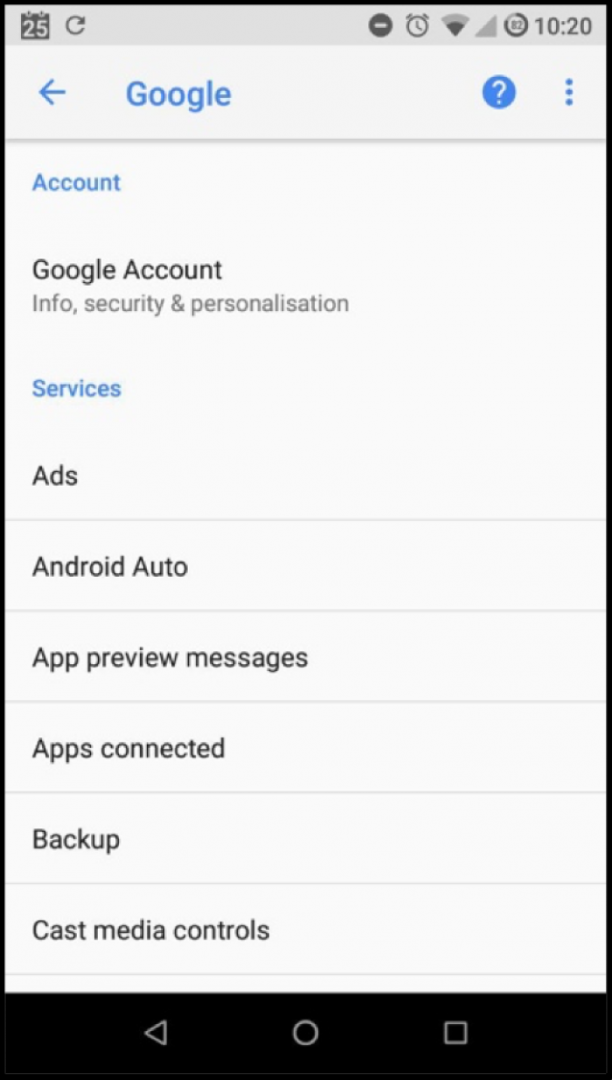The image showcases a smartphone screen displaying a webpage. The time on the phone reads 10:20, and the device shows a strong connection. At the very top of the screen, the word "Google" appears in blue, accompanied by a left-pointing arrow. Below this, there is a blue circle containing a question mark and a vertical trio of blue dots indicative of a menu or options list. 

The main content of the page is structured with several headers and sub-headers. The header "Account" is in blue, followed by the text "Google Account" in black. Directly beneath this, the section titles "Info," "Security," and "Personalization" are listed. 

Further down, another blue header reads "Services," under which various service options are listed in black text, including "Ads," "Android Auto," "App Preview Messages," "Apps connected," "Backup," and "Cast media controls."

At the bottom of the screen, the familiar navigation icons found on iPhones are visible: a left-pointing arrow, a home button, and a square, all set against a black stripe along the lower edge of the display. The overall design of the webpage is predominantly black and white, with the only color coming from the blue text and icons, giving it a very basic and plain appearance.